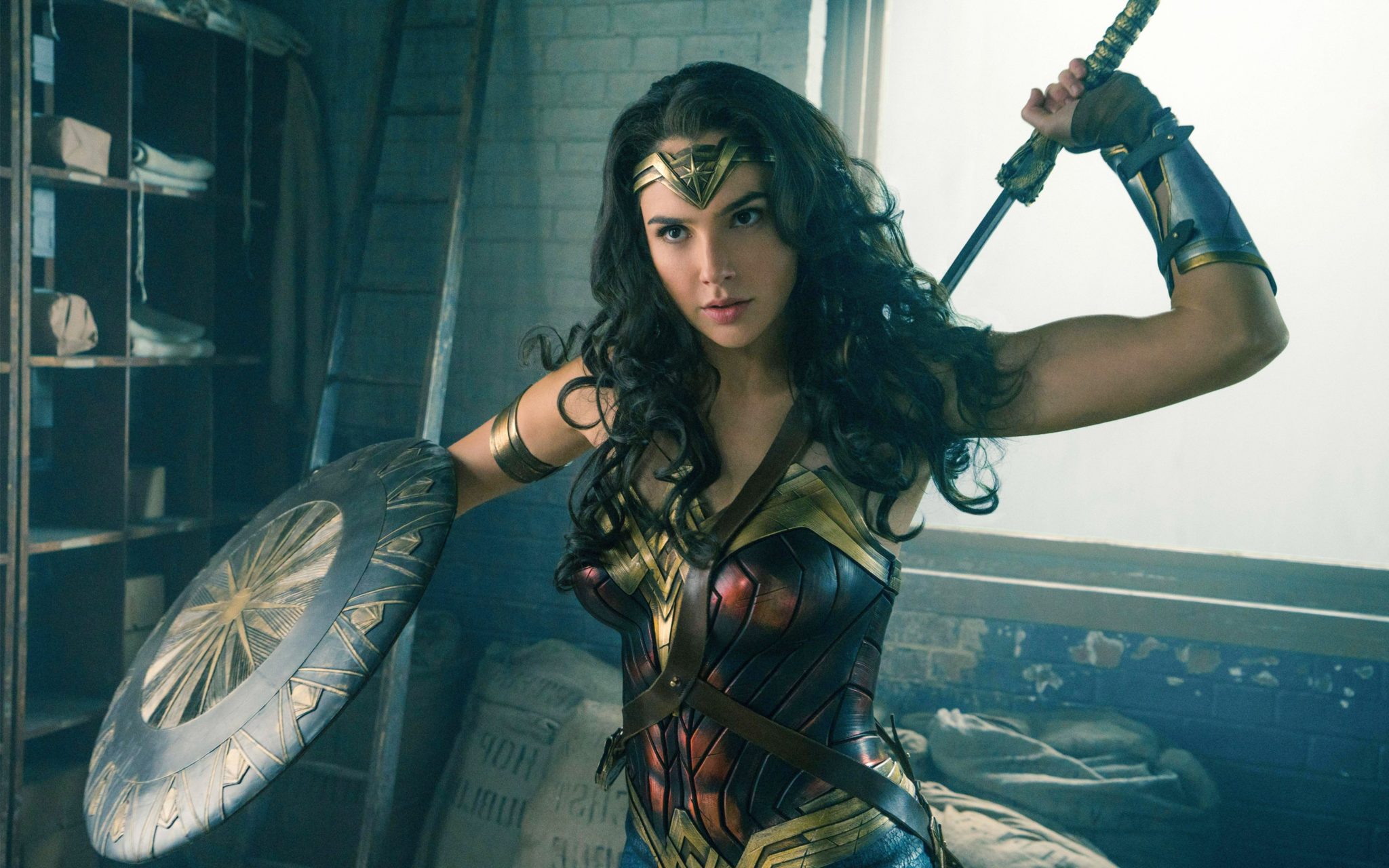In this detailed horizontal image, a realistic portrayal of Wonder Woman dominates the center of an indoor setting. She is depicted with long, dark, curly hair cascading to her shoulders and a tan complexion. She sternly gazes past the camera, her dark eyes brimming with intensity. Adorning her forehead is a golden headband, featuring a prominent star in the middle. Clad in her iconic superhero uniform, a blend of blue, brown, and golden hues, she exudes an aura of strength and readiness for battle. Her armor includes metal wrist guards lined with cloth and a gold armband on her right arm. In her left hand, she grips a black and gold shield, while her right hand draws a sword from behind her back.

The scene captures her from roughly the thighs up, highlighting her upper body and facial features. She stands inside an old-style room, untidy and filled with character. Behind her, a brick wall is partially visible, with a ladder leaning against it. To her left, numerous shelves and cubbies contain various items, adding detail to the room’s cluttered atmosphere. To the right, a window allows white light to flood in, casting an illuminating glow on Wonder Woman’s formidable stance.